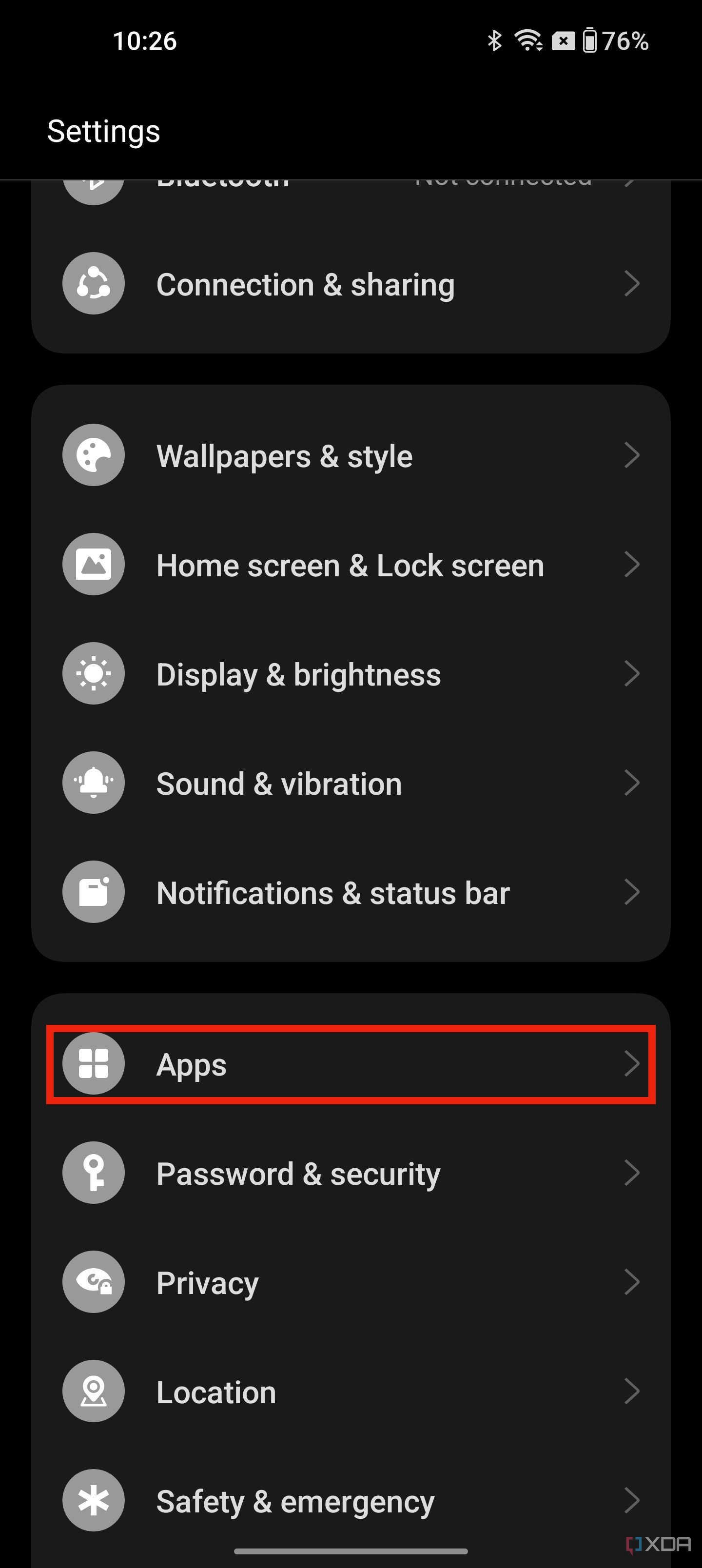In this image, the settings screen of a cell phone is displayed in great detail. At the top-left corner of the screen, the time is shown as 10:26. On the top-right corner, there are icons for Wi-Fi and battery status; the battery icon indicates that it is 76% charged. Immediately below, on the left-hand side, the word "Settings" is prominently displayed.

The screen is divided into visually distinct sections and subsections, each with a dark gray background separated by black horizontal dividers. At the very top, though not entirely visible in the image, there seems to be the title or name of an overarching category. Below this, the first visible category is "Connection and Sharing," each accompanied by an emblem to its left featuring a white design.

The second section includes several categories listed in the following order: "Wallpapers and Style," "Home Screen and Lock Screen," "Display and Brightness," "Sound and Vibration," and "Notifications and Status Bar."

The final section starts with an orange rectangle labeled "Apps," followed by categories labeled "Password and Security," "Privacy," "Location," and "Safety and Emergency." Across the bottom of the image is a horizontal gray line, marking the end of the settings list visible on the screen.